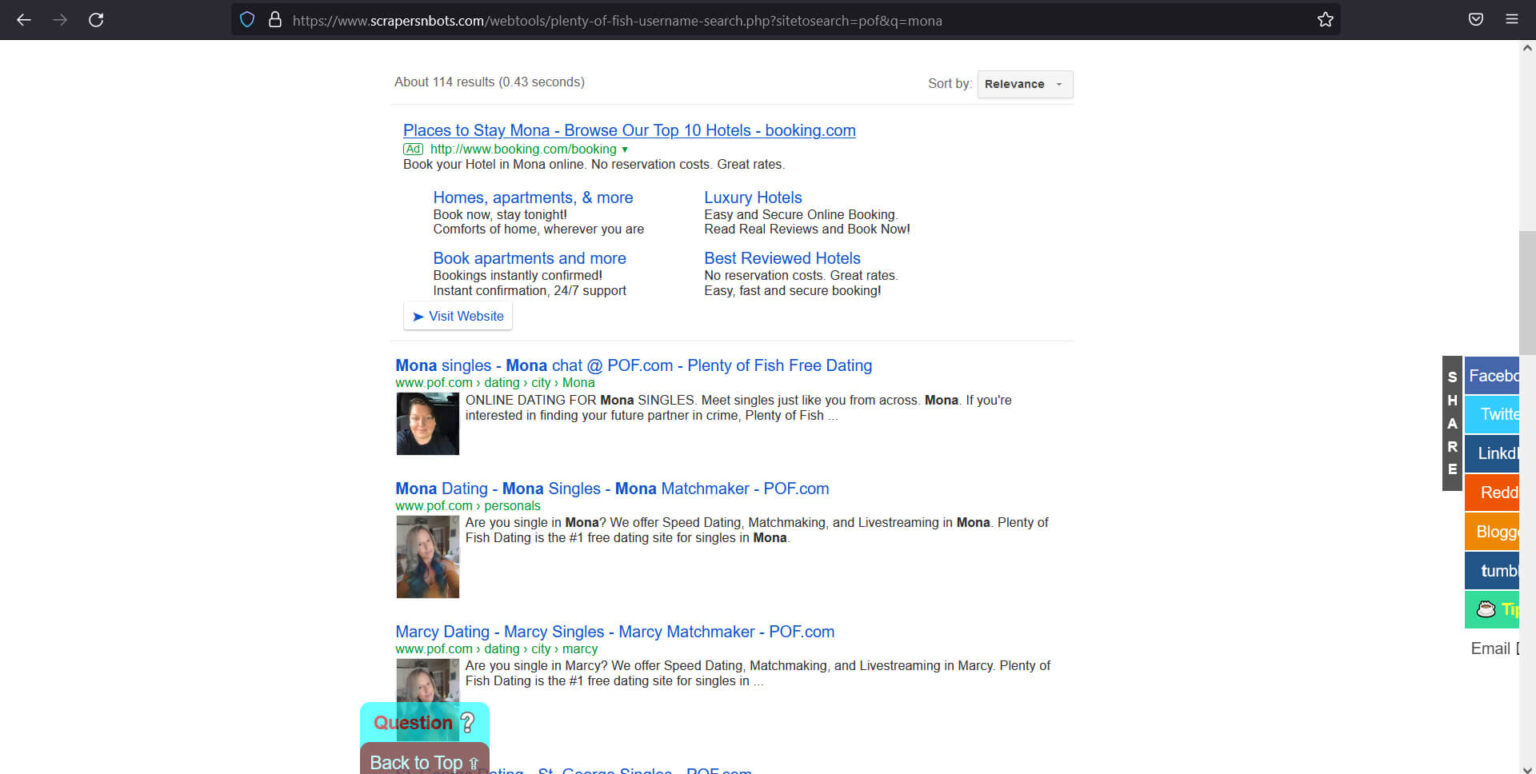This is an image of a webpage that is difficult to discern due to a prominent black bar obscuring part of it. The page background is very dark, making it challenging to read the details. At the top of the page, it displays "about one hundred and fourteen results" along with the search time in seconds, indicating search results for a particular query.

The first search result is titled "Places to stay Mona - Browse our top ten Hotels | Booking.com." It mentions homes, apartments, luxury hotels, and best-reviewed hotels. Below the title, there is a green URL text indicating it links to Booking.com.

The second result is titled "Mona singles | Mona chat | pdf.com." It references online dating platforms like Plenty of Fish and features an image of a woman. 

The third result is "Mona dating | Mona singles | Mona matchmaker | pdf.com" with another image of a different woman and references matchmaking services. Interestingly, the image of the woman appears the same as in the second result.

A fourth result mentions "Marcy dating | Marcy singles | Marcy matchmaker | pdf.com," showing a woman’s image, seemingly identical to the woman in the previous search result.

Additionally, there is a pop-up element with the word "questions" and a "back to top" option. 

On the right side of the page, there are several share buttons for social media platforms including Facebook, Twitter, LinkedIn, Reddit, Blogspot, Tumblr, and one indistinct icon that might be WhatsApp. The page layout and visual elements make it difficult to fully grasp all the content.